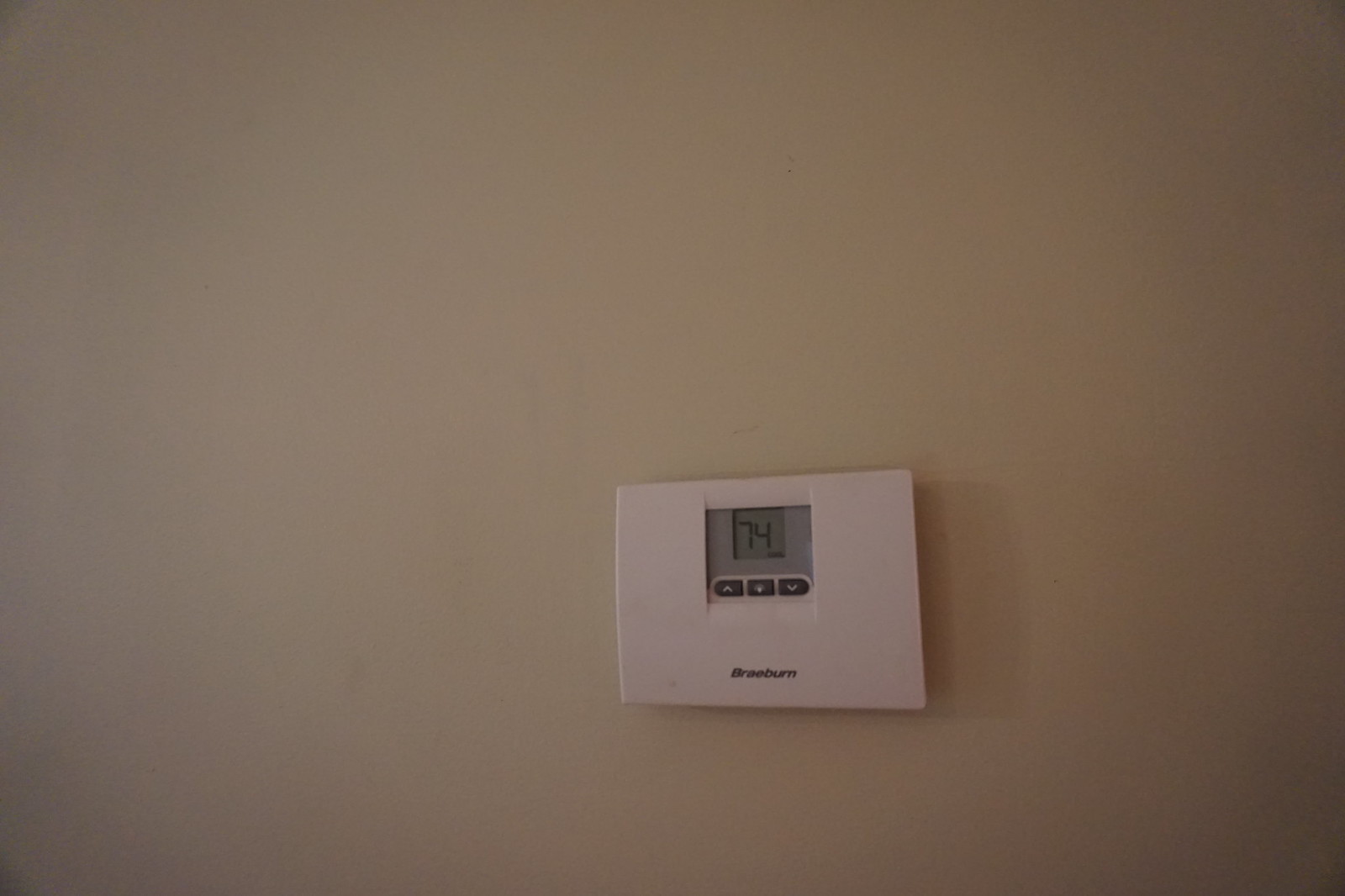On a light pinkish-brown wall, positioned towards the bottom right, there is a rectangular plastic thermostat with a subtle pink hue. The thermostat has "Brass Burn" inscribed in dark gray letters. Dominating the center of the device is a large window featuring a smaller, clear window within, displaying the current temperature of 74°F. Within the larger window, there are three dark gray buttons at the bottom: one with a white up arrow, another with a white down arrow, and the third likely labeled as an off button. This neat, functional thermostat contrasts gently with the soft-toned wall.